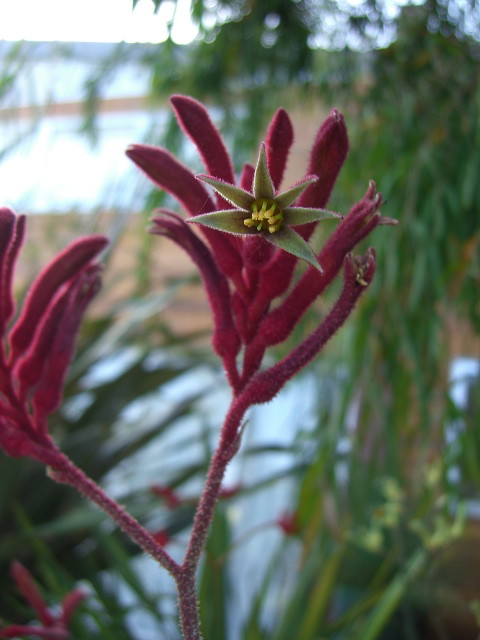This photograph captures an exotic and unusual plant with a vivid maroon, crimson, or dark fuchsia hue. The main stem, which is pinkish and appears covered in fuzzy spore-like needles, ascends and splits into two branches. The right branch further bifurcates several times into bud-like structures resembling slender, purple fingers reaching out. At the center top of the plant is a striking green flower, reminiscent of an aloe, with a starfish-like appearance. The green petals house yellowish-green stamens and anthers. The blurred background hints at abundant green foliage, including possibly tall grass or tree branches, and suggests the presence of a body of water, giving the scene a swampy or delta-like ambiance.